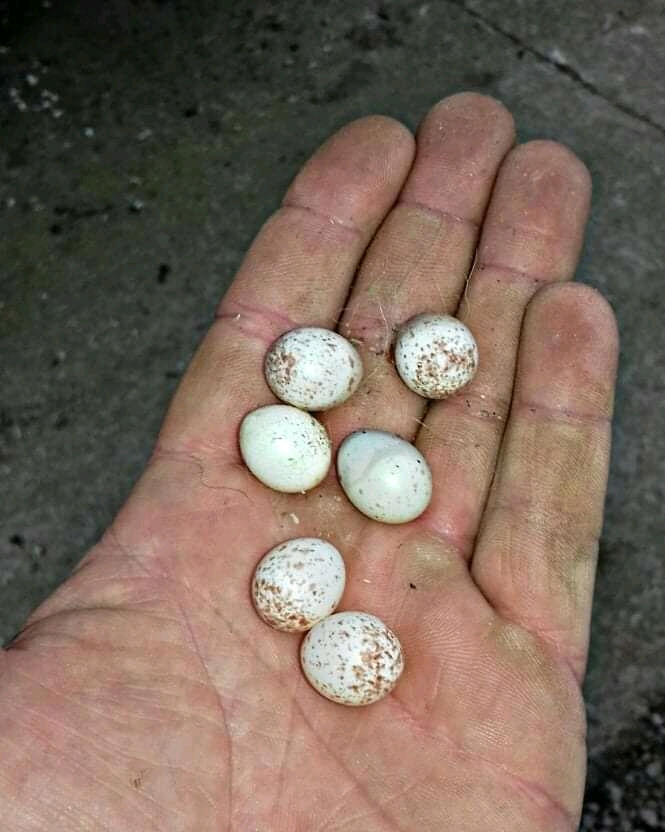In this color snapshot, a close-up shot captures the open, calloused palm and the top four fingers (thumb not visible) of an older, white person's very dirty hand. Cradled within the hand are six tiny eggs, each roughly an inch long and an inch wide. These eggs are predominantly white with irregular brown speckles randomly scattered across their smooth, slightly oval shells. The eggs have not hatched yet. The palm and fingers of the hand are heavily lined and soiled with dirt, featuring noticeable calluses, red marks, and even a cut on one of the fingers. The background depicts a ground surface resembling a sidewalk or driveway, with patches of dirt, white rocks, and gray pebbles visible.